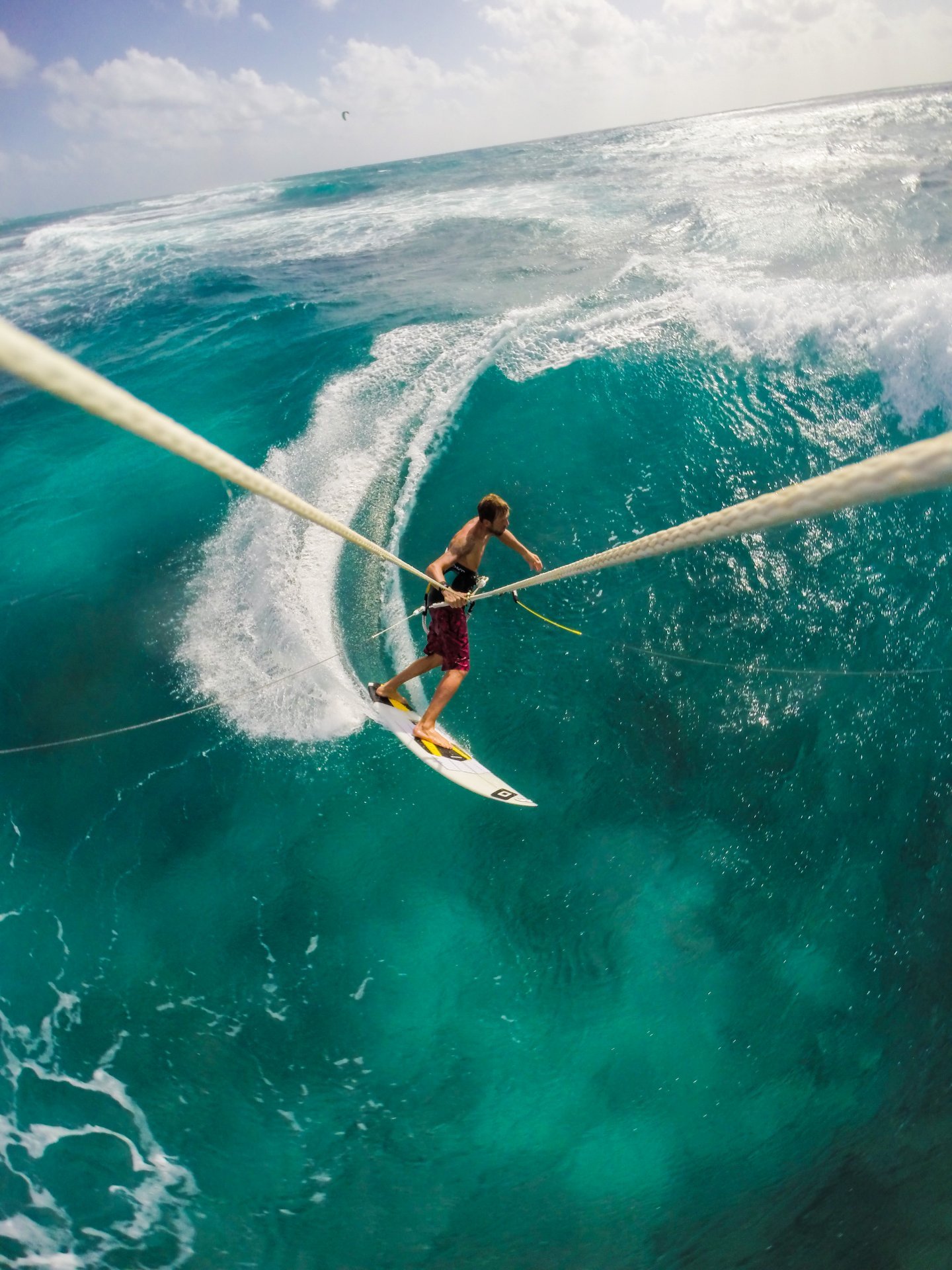In this vibrant outdoor photograph, a young man is captured mid-windsurf, navigating the turquoise waters that shimmer under the sunlight. He wears red swim trunks and firmly stands on a white surfboard adorned with yellow grip pads. The clear, bluish-green ocean below presents an almost translucent depth, akin to the picturesque waters of the Caribbean or Baja, California. The windsurfer is connected to a set of ropes that stretch upward, likely attached to a sail, though the sail itself is not visible in the image. His right hand clutches one of the ropes while his feet remain steadfast on the board. The dynamic perspective, seemingly from a camera mounted above, offers a stunning bird's-eye view of the scene. The ocean's surface is dotted with white caps, indicating a slightly rough sea, and the trail of white waves left in his wake adds a sense of motion. Above, the sky is a rich blue, scattered with fluffy white clouds, completing the idyllic seascape.